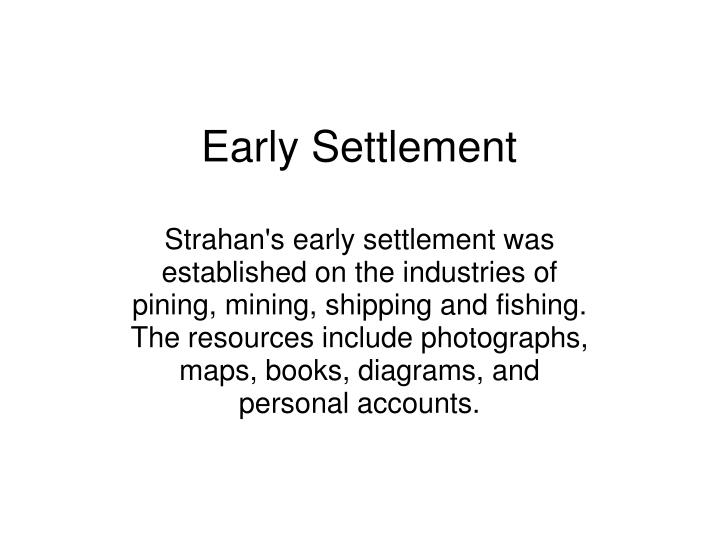The image depicts an informational slide set against a plain, white background, featuring black text centrally aligned. At the top-center of the slide, the title reads "Early Settlement." Below the title, a paragraph explains that "Strahan's Early Settlement was established on the industries of pining, mining, shipping, and fishing." Additionally, it mentions that resources related to this topic include photographs, maps, books, diagrams, and personal accounts. The slide's design suggests it could be part of a PowerPoint presentation or an informational blurb, with no other objects or colors present.